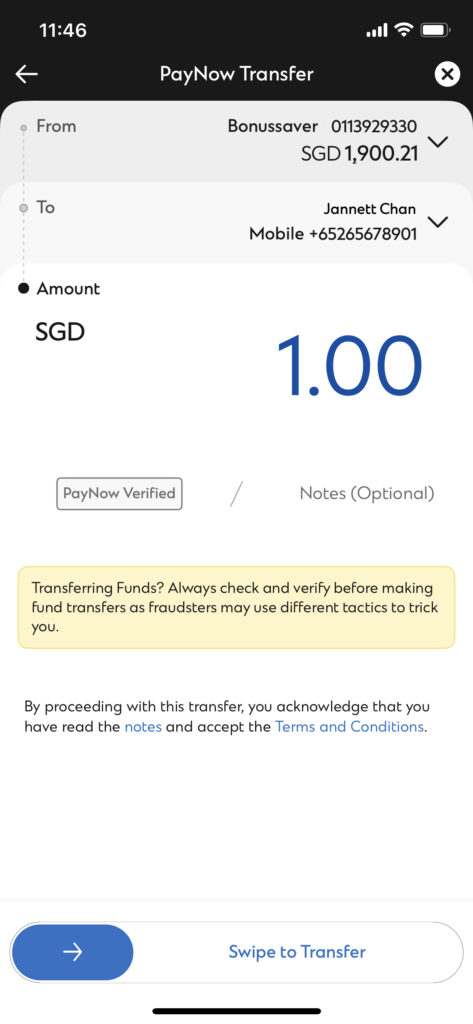**Detailed Caption:**

This screenshot depicts a digital interface for a paint-out transfer transaction. At the very top, the screen has a black background with white text displaying "PAINT-OUT TRANSFER." On the left-hand side, the time "11:46" is visible, while the right-hand side shows symbols indicating full carrier signal, full Wi-Fi, and full battery status.

Centered below the title is a white left-pointing arrow. Beneath this, the phrase "Paint-Out Transfer" is prominently displayed. Adjacent to this text is a white circle containing a black "X."

The main content area begins with a medium gray tab labeled "From" on the left. It indicates the source account "Bonus Saver 0113929330," with a balance of "SGD $1,900.21." Below this, a light gray section contains an arrow pointing downward, a small gray dot next to the word "To," specifying the recipient "Janet Chan," and her mobile number "+652-656-78901." The transfer amount to Janet Chan is "SGD $1."

Further down, the screen states "Paint-out verified," clarifying the transaction's legitimacy. A message follows, warning users about the risks of fraudulent activities and advising verification before transferring funds.

Below this, a white box with a gray outline contains the instructions "Notes (Optional)" in gray text. A yellow box underneath provides a cautionary note: "Transferring funds. Always check and verify before making fund transfers as fraudsters may use different tactics to trick you."

The lower section features a message on a white background: "By proceeding with this transfer, you acknowledge that you have read the notes and accept the terms and conditions," with the words "notes" and "terms and conditions" highlighted in blue text. 

Finally, at the bottom, a faint gray line separates the instruction "Swipe to Transfer," displayed within a white oval with a blue gradient oval on the left and a right-pointing white arrow. The screen concludes with the short black line typical at the bottom of phone screens.